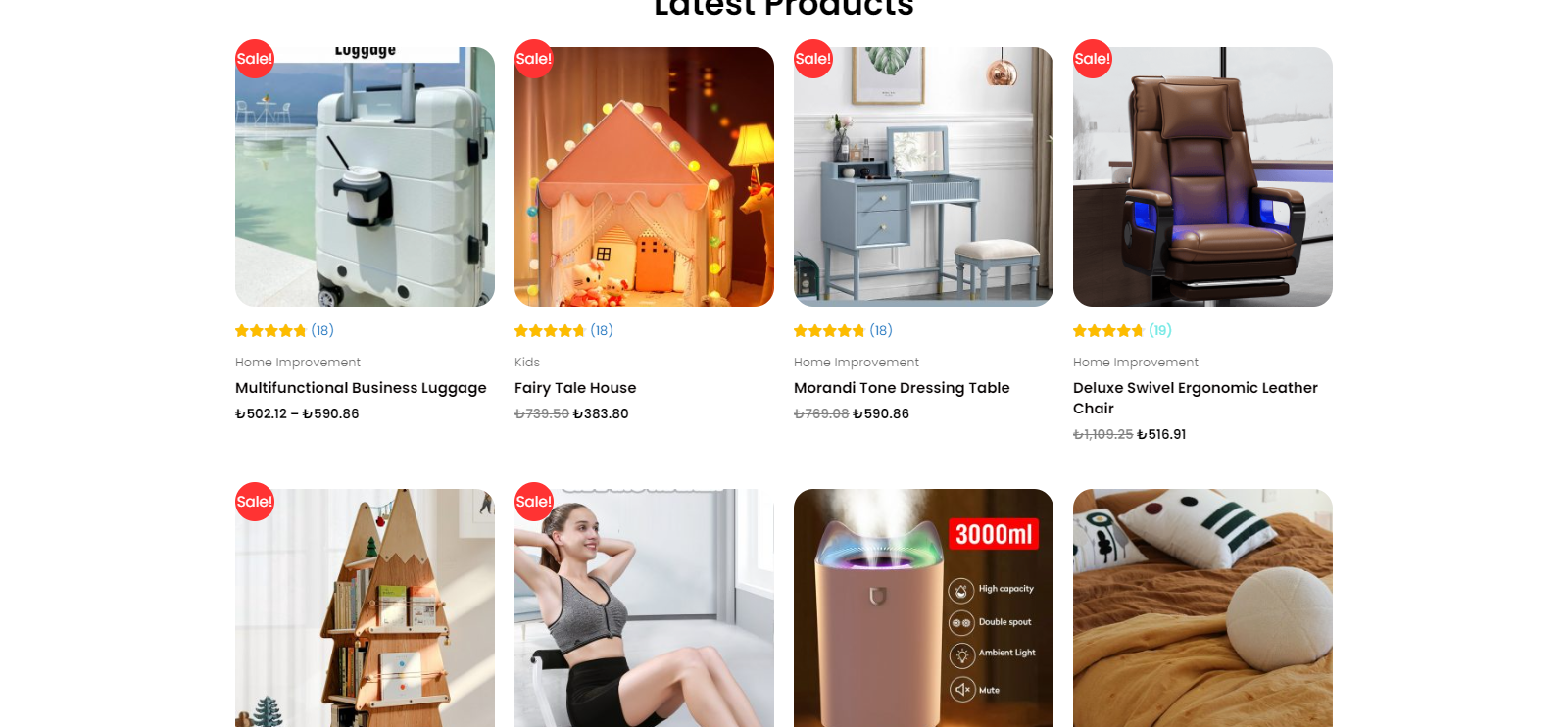**Caption:**

On a white background, the top portion of the image features partially cut-off black letters spelling out "latest products." Below this, the image is divided into two rows of four product images each. The top row is fully visible, while the bottom row is partially cut off.

- **Top Left Image:** This picture showcases a white, hardbound suitcase set against the backdrop of a pool with mountains and a blue sky. A red circle with white letters indicating "SALE" is superimposed on the image. Above the suitcase, the text "Luggage" appears in black letters. Underneath, it has a star rating of 4.5 out of 5 stars, with the number "(16)" in blue parentheses. Directly below, in faint black letters, are the words "home improvement," followed by larger black letters reading "Multifunctional Business Luggage." The price is given as "50212-59086" in an unfamiliar currency.

- **Top Center Left Image:** Depicts an interior scene that resembles a whimsical fairy house. The dimly lit room is outlined with various round lights and contains yellow and orange pillows, as well as Hello Kitty stuffed animals. A lamp is positioned toward the upper center right. This product has a star rating of 5 out of 5 stars, though the number in gray parentheses is unreadable. Below, in black letters, it says "Fairy Toll House," and a gray, crossed-out price is followed by a new price of "383-80" in another currency.

- **Top Center Right Image:** Features a well-lit room with a grayish-white wall, part of a picture frame, and light blue furniture including a desk, a cushioned seat, and possibly other items. It has a 5 out of 5 star rating with "(18)" in blue parentheses. The category "home improvement" is present in gray letters, followed by "Marodi Trone Dressing Table" in black letters. The previous price in small gray letters is crossed out, with a new price of "590-88" in an unfamiliar currency.

- **Top Right Image:** Displays a long, comfortable-looking brown leather chair with white-framed windows in the background. It also has a 5 out of 5 star rating, though the number in aqua parentheses is too small to read. Below, gray letters spell out "home improvement," followed by "Deluxe Swivel Ergonomic Leather Chair" in black letters. The original price is crossed out in gray, with a new price of "516.51" in another currency next to it.

The bottom row, cut off at the descriptions, includes:

- **Bottom Left Image:** A bookcase shaped like mountains with a gray side and jagged white areas representing snow and books on the shelves. The room is well-lit, possibly with a window behind the bookcase.

- **Bottom Center Left Image:** A Caucasian woman doing sit-ups in a well-lit gray room. She wears black shorts, a gray bra top, and has short black hair tied in a ponytail.

- **Bottom Center Right Image:** Shows a pink cylindrical device emitting steam against a brown background. At the upper right, there is a red rectangle with white letters reading "3000 ml" and smaller white icons and text underneath.

- **Bottom Right Image:** Features a tan bedspread on a bed with three pillows. One pillow is circular and white, while the other two are square with black decorations, including stripes and dots, against a white background.